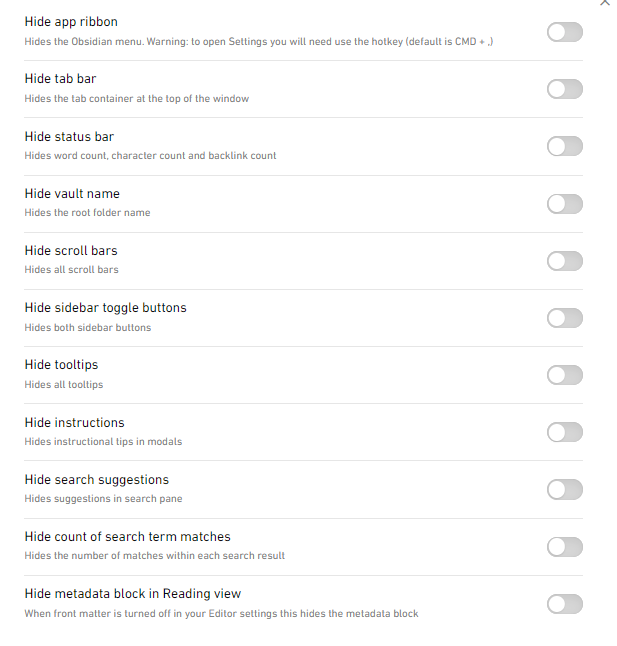This screenshot captures the customization section of a website interface. The page displays a list of over ten settings, each designated with a specific function and equipped with a toggle button on the right side for user interaction. The options listed are mainly focused on visibility settings within the website’s interface.

1. **Hide App Ribbon:** Toggle switched off.
2. **Hide Tab Bar:** Toggle switched off.
3. **Hide Status Bar:** Toggle switched off.
4. **Hide Value Name:** Toggle switched off.
5. **Hide Scroll Bar:** Toggle switched off.
6. **Hide Sidebar Toggle Buttons:** Toggle switched off.
7. **Hide Tooltips:** Toggle switched off.
8. **Hide Instructions:** Toggle switched off.
9. **Hide Search Suggestions:** Toggle switched off.
10. **Hide Count of Search Term Matches:** Toggle switched off.
11. **Hide Metadata Block in Reading View:** Toggle switched off.

At the top right corner of the interface, there is an up arrow situated above the toggle buttons. Each section is separated by a horizontal line, and beneath each option is a brief explanatory phrase that details the purpose of the setting. This layout provides a clear and organized means for users to customize various aspects of their website experience.